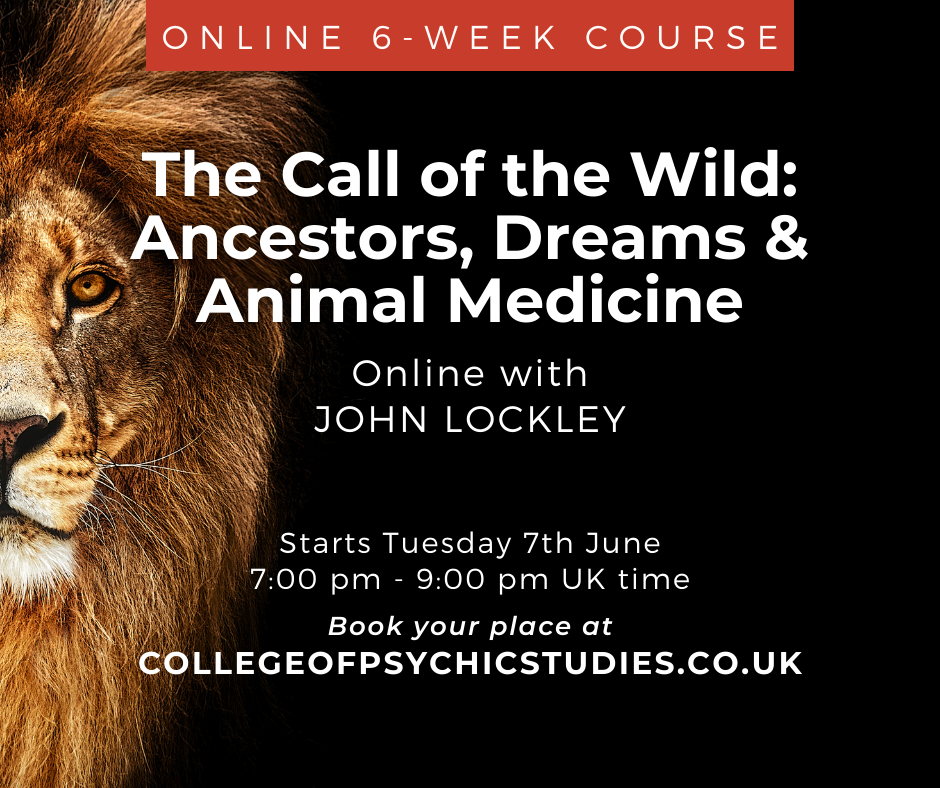This image is an advertisement for an online course with a black background that prominently displays half of a lion's face on the left side. The lion, with striking golden-brown eyes, a brownish nose, white whiskers, and a yellow-brown mane, looks intently towards the viewer. The text on the advertisement is in white and stands out sharply against the dark backdrop. At the top, a red banner announces an "Online Six-Week Course." Below, the main text reads, "The Call of the Wild: Ancestors, Dreams, and Animal Medicine," followed by "Online with John Lockley." The course details specify that it starts on Tuesday, 7th June, from 7pm to 9pm UK time. Viewers are directed to book their places at www.collegeofpsychicstudies.co.uk.